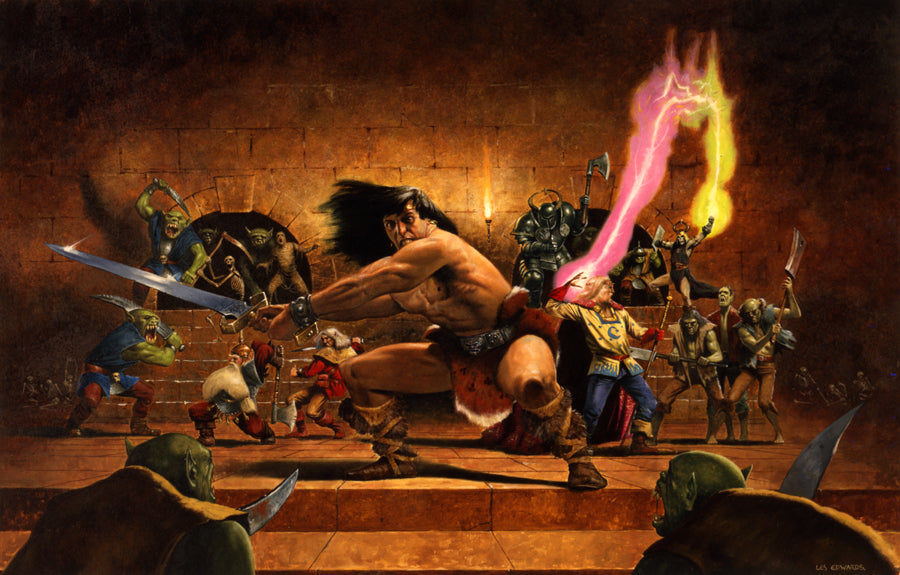In the computer-generated artwork, a colossal human warrior or barbarian takes center stage in an intense indoor battle scene. Shirtless and donning a red fabric loincloth with a belt and brown boots, he crouches low to the ground, his long black hair blowing to the left. His muscular arms extend to the left, wielding a massive silver sword with a gold handle. This sword is poised above two green orcs with visible backs, shoulders, and heads at the bottom of the image, both brandishing knives or swords. The indoor setting is vividly constructed from brown bricks and stone, bolstering the atmosphere of the conflict.

Behind the warrior, a fierce skirmish unfolds. On the left, a green orc wields a sword against a dwarf with a lush white beard, while more orcs loom in the background. To the right, a wizard in blue pants and a yellow shirt casts a striking pink beam of magic from his hand, while another character channels a bright yellow beam. These detailed spell effects add dynamic color to the scene.

Further into the background, two curved entryways atop stone steps spill forth additional warriors, contributing to the bustling chaos. The overall scene captures a vivid, action-packed moment of a grandiose battle, rich with fantastical creatures and magical elements amidst a rugged, stone-walled environment.